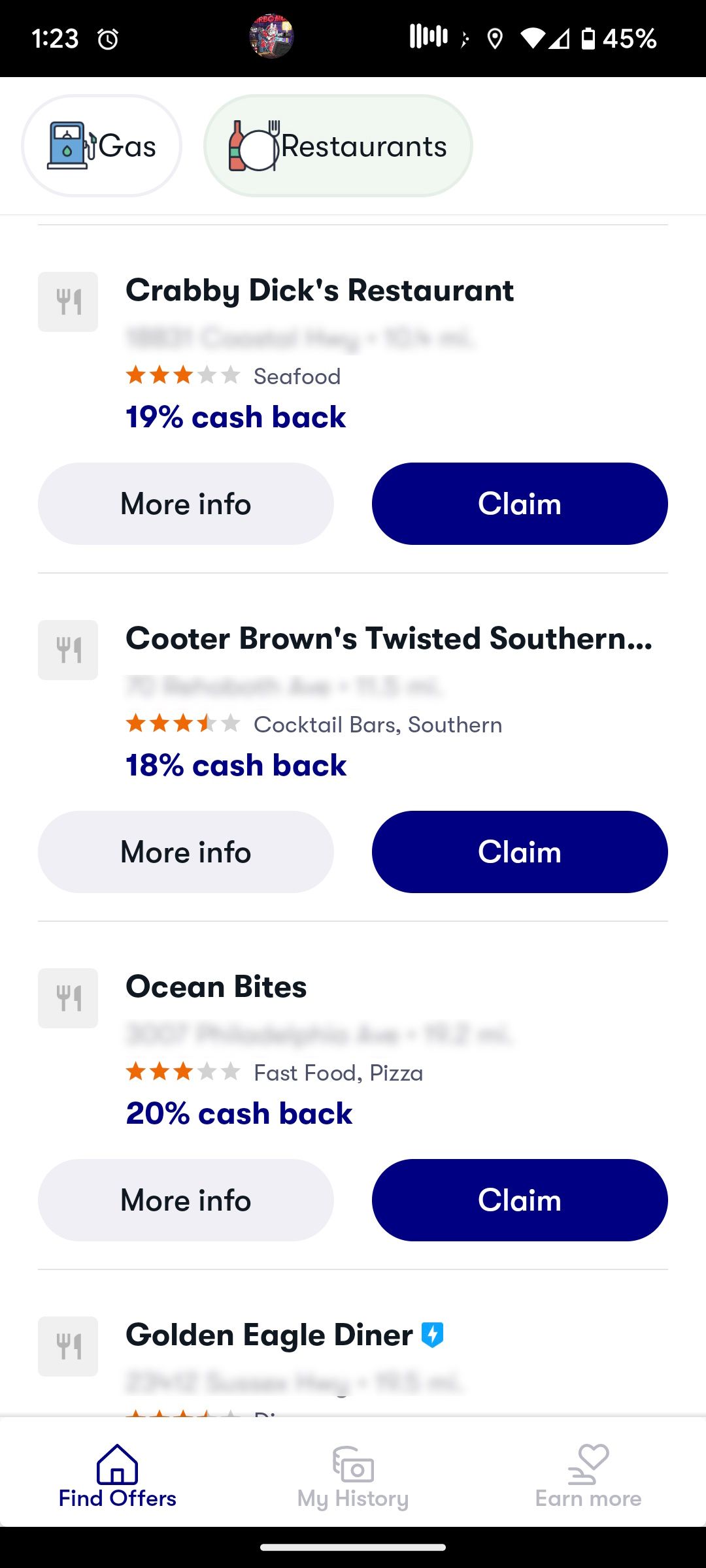Screenshot of a Phone Displaying a Restaurant Search:

The image is a screenshot taken from a smartphone. At the top, the screen displays a black background, overlaid with white text. On the top left, the current time is shown as 1:23. On the top right, the battery level is indicated to be at 45%. Beneath this status bar, the user appears to be conducting a search for restaurants within a certain app.

The interface includes a navigation section with circular icons; the first icon is labeled "Gas," and the second is labeled "Restaurants." Further down, a list of restaurant options is displayed, each with specific details.

1. **Krabby Dick's Restaurant**:
   - The address is blurred out.
   - Rated 3 stars.
   - Categorized as a seafood restaurant.
   - Offers 19% cash back.
   - Options to view more info or claim a deal.

2. **Cooter Brown's Twisted Southern**:
   - The full address is cut off.
   - Rated 3.5 stars.
   - Offers 18% cash back.
   - Options to view more info or claim a deal.

3. **Ocean Bites**:
   - Rated 3 stars.
   - Specializes in fast food pizza.
   - Offers 20% cash back.
   - Options to view more info or claim a deal.

4. **Golden Eagle Diner**:
   - Further details are not visible in the screenshot.

At the bottom of the screenshot, a black line runs across the screen, likely part of the phone’s interface or a visual separator within the app.